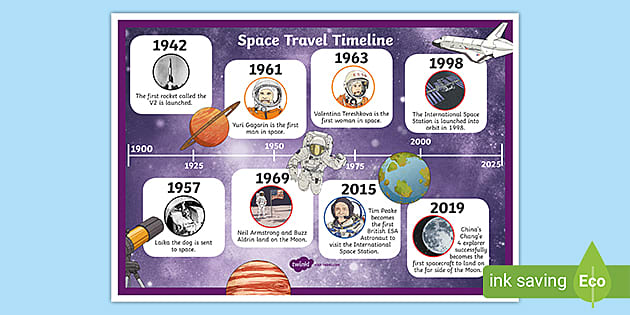Set against a light blue background, this rectangular-shaped image features a central poster dedicated to a "Space Travel Timeline." The poster itself has a prominent purple background and its content is organized within a white-bordered, horizontal layout. At the top center of the poster, "Space Travel Timeline" is labeled in white text. The timeline spans different years with significant space travel events, presented in a sequence of eight white squares, each containing a year, an illustration, and descriptive text.

The years highlighted are 1942, 1957, 1961, 1963, 1969, 1998, 2015, and 2019. Each square features detailed drawings such as astronauts, planets, spaceships, and telescopes. Notable events include the 1942 launch of the first rocket V2, Yuri Gagarin becoming the first man in space in 1961, Valentina Tereshkova's 1963 achievement as the first woman in space, and Neil Armstrong and Buzz Aldrin's 1969 moon landing. It also records Laika the dog's 1957 space journey, the International Space Station's 1998 deployment, the first British ESA astronaut's 2015 visit to the ISS, and China's successful 2019 landing on the moon's far side.

Additionally, at the bottom right corner of the image, there's a green-background rectangle with a leaf design that reads "ink saving eco," emphasizing an environmentally conscious theme.